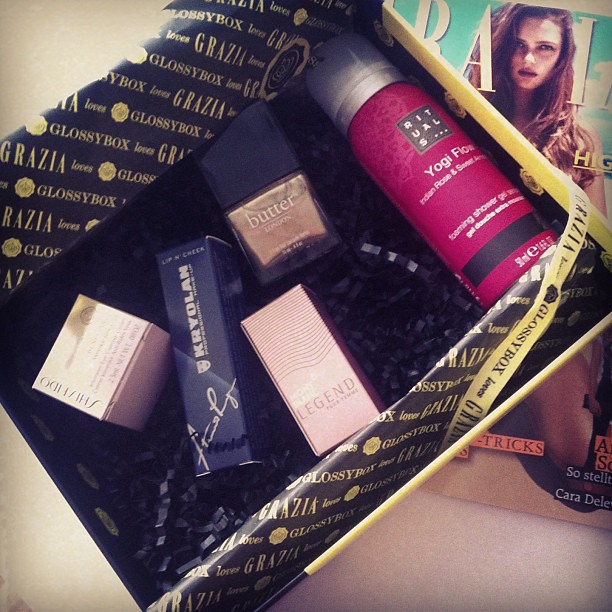This color photograph captures an overhead view of an open, glossy yellow box containing various beauty products, framed against a partial magazine cover that features a young girl looking towards the camera. The interior of the box is lined with yellow and black tissue paper along with blue and black confetti padding. At the forefront, the box holds five distinct beauty items. The first is an enigmatic small pink cube. Next to it, there’s a rectangular package labeled "KRYOLAN lip color, lip, and cheek color." Beside this is a small pink cardboard box inscribed with "Legend." Positioned above it is a square-shaped glass container with "butter" and "foundation" mentioned, suggesting it contains a type of makeup foundation. Lastly, there’s a small red metal canister with "Yogi flow, Indian rose, and sweet foaming shower gel." The bright colors of the items—yellow, dark blue, light pink, beige, tan, orange, and teal—stand out vividly against the confetti and tissue paper, creating an appealing aesthetic. The angle of the photograph, taken slightly askew from directly overhead, emphasizes the arrangement of the products and the detailed textures within the box.